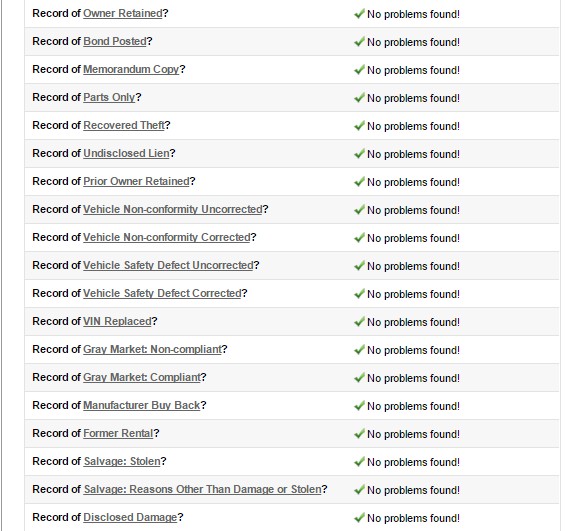The image displays a comprehensive report detailing various records associated with the vehicle, each accompanied by an underlined label and a green checkmark indicating no issues found. The highlighted labels include: 

- Owner Retained 
- Bond Posted 
- Memorandum Copy 
- Parts Only 
- Recovered Theft 
- Undisclosed Lien 
- Prior Owner Retained 
- Vehicle Non-Conformity Uncorrected 
- Vehicle Non-Conformity Corrected 
- Vehicle Safety Theft Uncorrected 
- Vehicle Safety Theft Corrected 
- VIN Replaced 
- Gray Market Non-Complaint

Each item to the right signifies "no problems found," affirming the vehicle's clear status across all these categories.